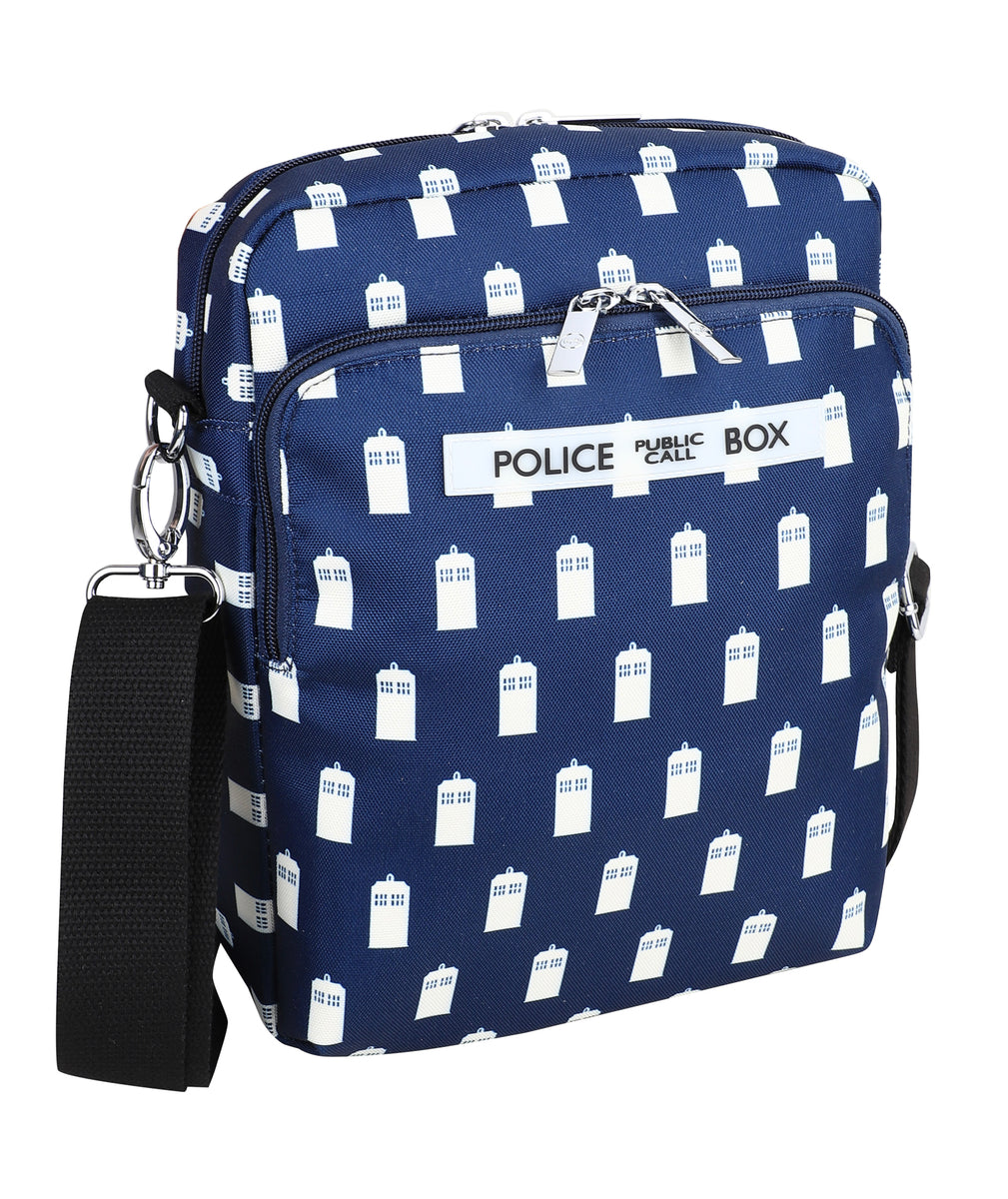This detailed product image showcases a Doctor Who-themed backpack, meticulously designed in dark navy blue canvas fabric adorned with a repeating pattern of white public call boxes, a clear nod to the iconic TARDIS from the series. The backpack features a prominent label on the front pocket with "Police Public Call Box" written in black lettering on a white background. This compact yet spacious accessory includes two main zippered compartments: a large main section capable of holding items such as a 17-inch laptop, and a smaller front pocket. Both compartments are equipped with dual silver zippers that meet in the center. The bag also includes a black woven strap attached by metal clasps on either side, which can be used to carry the backpack on your wrist or as an additional handle. With its detailed Doctor Who graphics and practical design, this backpack is perfect for fans of the franchise looking for a blend of style and functionality.